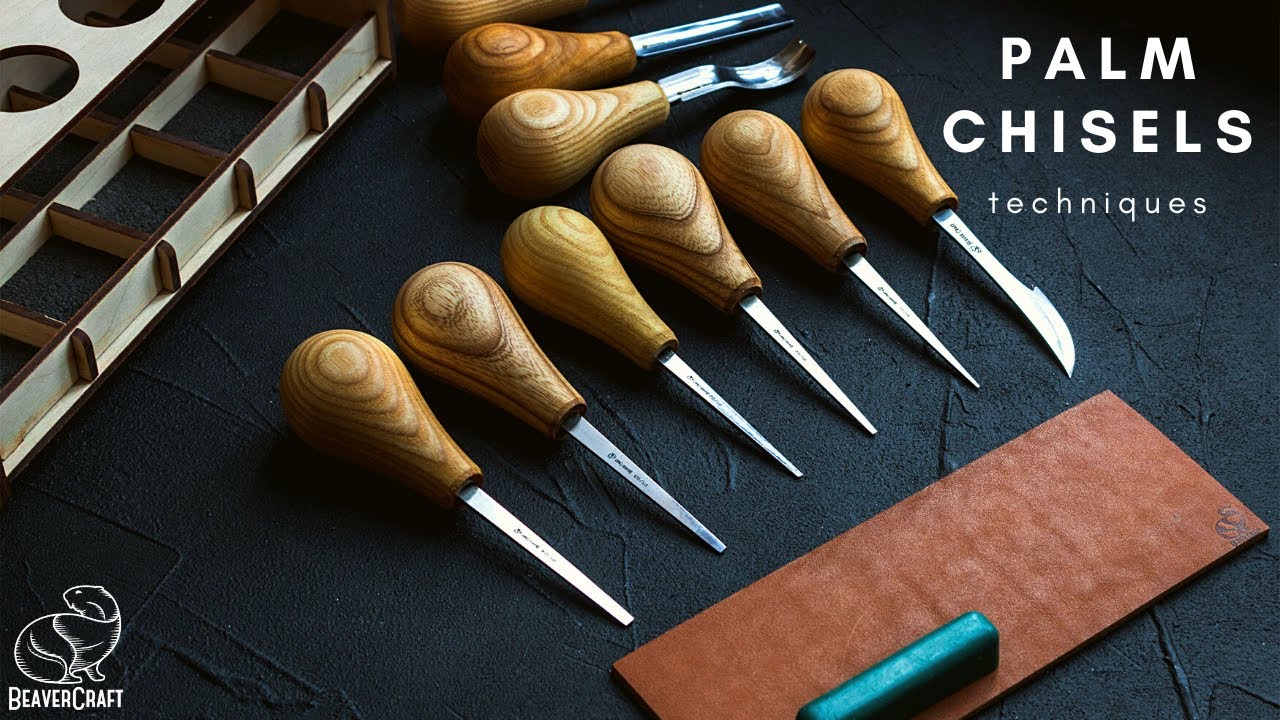The image is an advertisement showcasing a collection of woodworking chisels. In the upper right corner, white text reads "Palm Chisels Techniques." The chisels, each with a distinct wooden handle featuring a natural wood grain pattern, are arranged on a black surface. There are eight chisels clearly visible, with another one partially seen. These chisels have sharp metallic tips, with one resembling a knife. On the bottom left is the branding "Beaver Craft" accompanied by a white outline logo of a beaver. In the bottom right corner, a small brown block with a green component is present. In the upper left, a white and brown wooden structure is partially visible, likely related to the chisels' use. The consistent design elements and positioning suggest a clear and professional presentation aimed at woodworking enthusiasts.